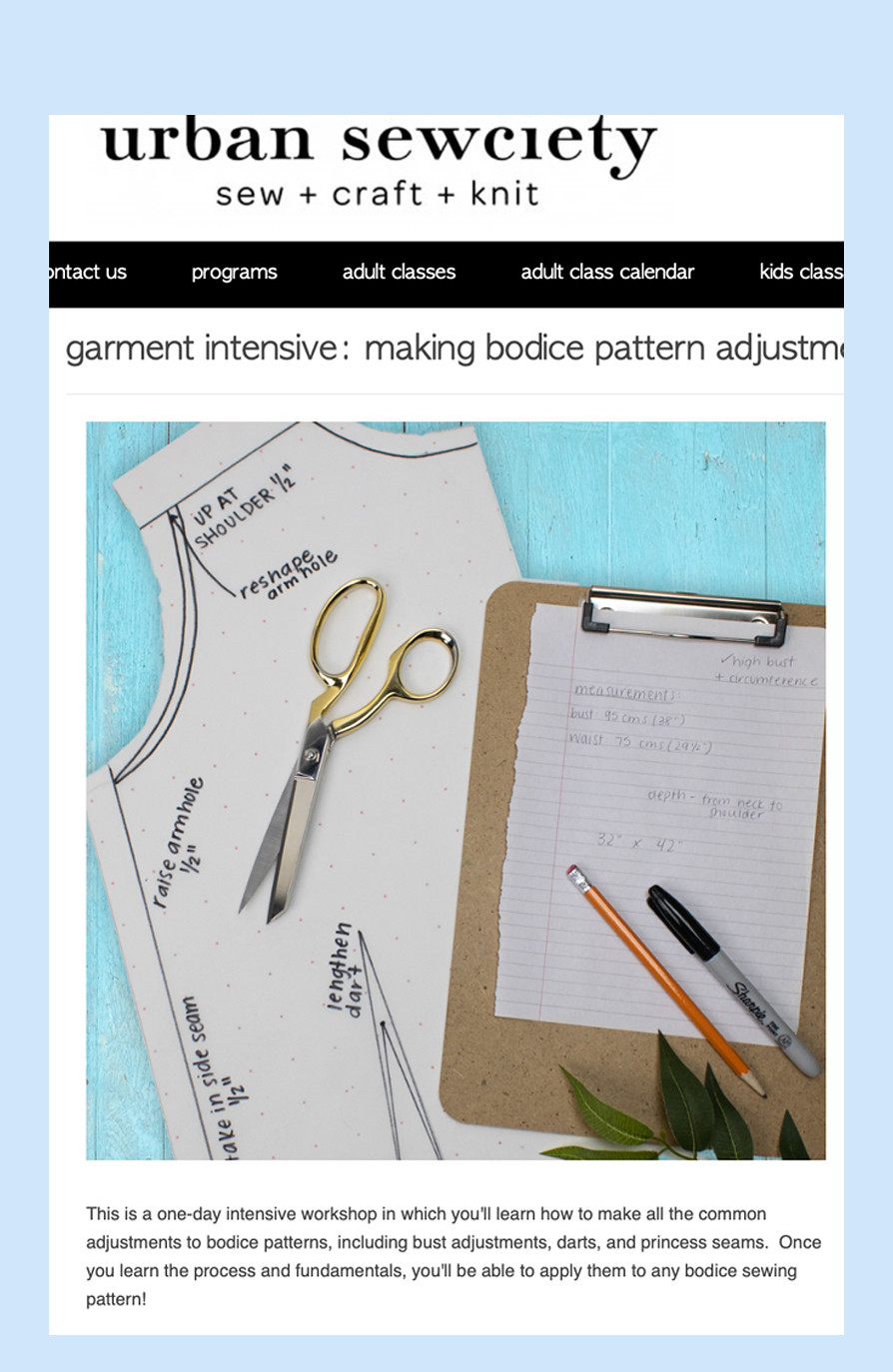The image is a detailed screenshot of a webpage for Urban Society, spelled "S-E-W-C-I-E-T-Y," featuring a header in a serif black font on a white background. The page is bordered by a blue rectangular frame. Just below the header, in a sans-serif font, the motto "Sew plus Craft plus Knit" is displayed. Directly beneath this, a black navigation bar with white text provides menu options: "Contact Us," "Programs," "Adult Classes," "Adult Class Calendar," and "Kids Classes." 

The main content announces a workshop titled "Garment Intensive: Making Bodice Pattern Adjustments" and showcases a real-life image. This central photo highlights a sewing pattern with labels like "Up at Shoulder," "Reshape Armhole," and "Raise Armhole," placed alongside a pair of gold and silver scissors. To the right, there is a brown clipboard holding a white-lined paper featuring measurements, accompanied by a black Sharpie and a pencil.